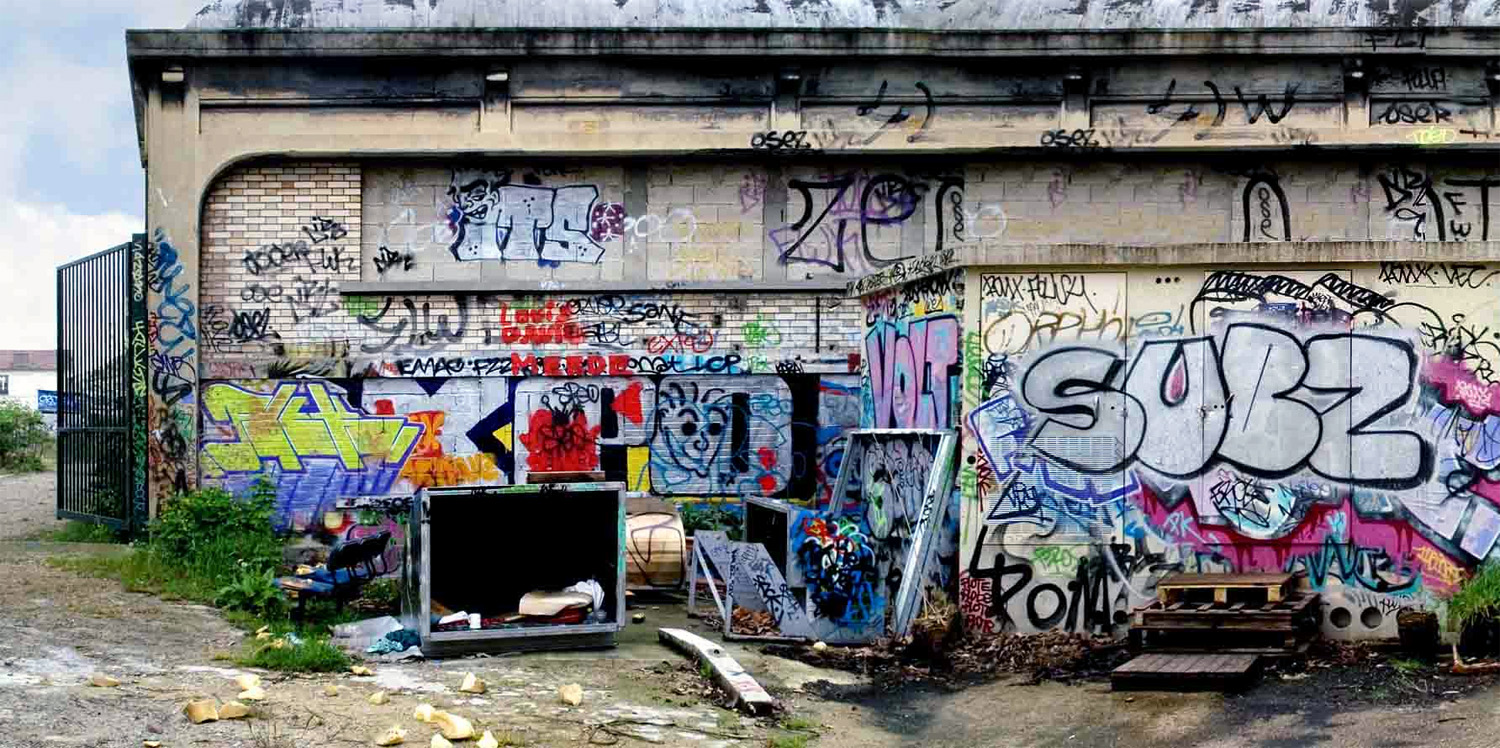The image captures a large, decrepit building that appears to be abandoned. The primary focus is a sizable brick and concrete structure heavily adorned with vibrant graffiti in various neon and bright colors. The front of the building reveals extensive grime, mildew, and chipping paint, particularly around the roof, with dirt patches and graffiti featuring an array of styles from letters to faces, including "S-U-B-Z" in bubble writing and other tags in red, teal, magenta, and neon green. Below the graffiti, the scene transitions into a neglected lot filled with scattered garbage, including tipped-over garbage cans, metal frames, and wooden pallets also marked with graffiti. Rocks and miscellaneous debris litter the area, with small patches of green weeds adding to the overall dilapidated feel. On the left edge of the image, a black metal gate leading further down what once may have been a driveway or parking lot stands ajar, reinforcing the sense of abandonment.